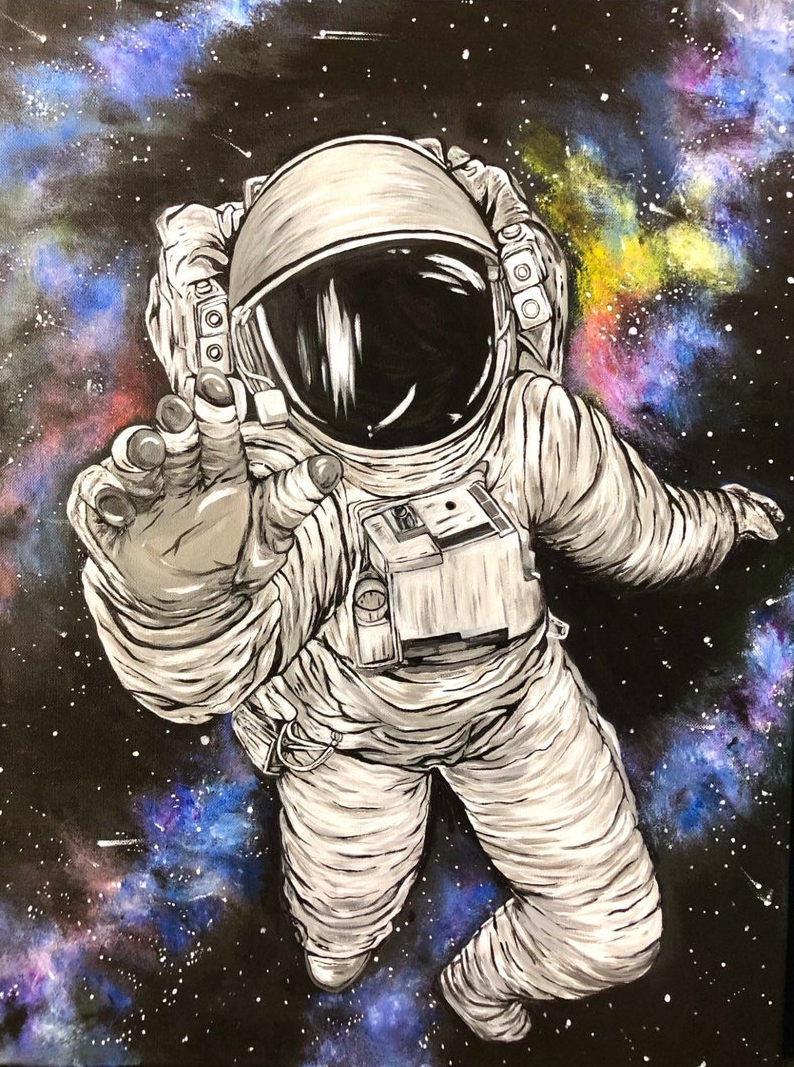This image is a detailed, cartoon-like drawing of an astronaut floating freely in the depths of outer space, with no tether visible. The astronaut is dressed in a white space suit, reminiscent of mummy wrappings, with a distinctive, dark black face shield obscuring the face entirely. The left hand of the astronaut is positioned directly toward the viewer, while the right arm is outstretched with the hand open, and the left arm is slung backward.

The background is a stunningly colorful depiction of outer space, featuring a rich tapestry of orange, yellow, and purple clouds, particularly prominent on the right side of the astronaut's helmet. The sky itself is a deep, star-studded black, interspersed with vibrant hues that resemble a watercolor painting in a striping pattern. These bright streaks of color evoke the cosmic beauty of nebulae or galaxies, adding an ethereal quality to the scene. There are no textual elements or insignia on the astronaut's suit, giving a universal, borderless aspect to the image.